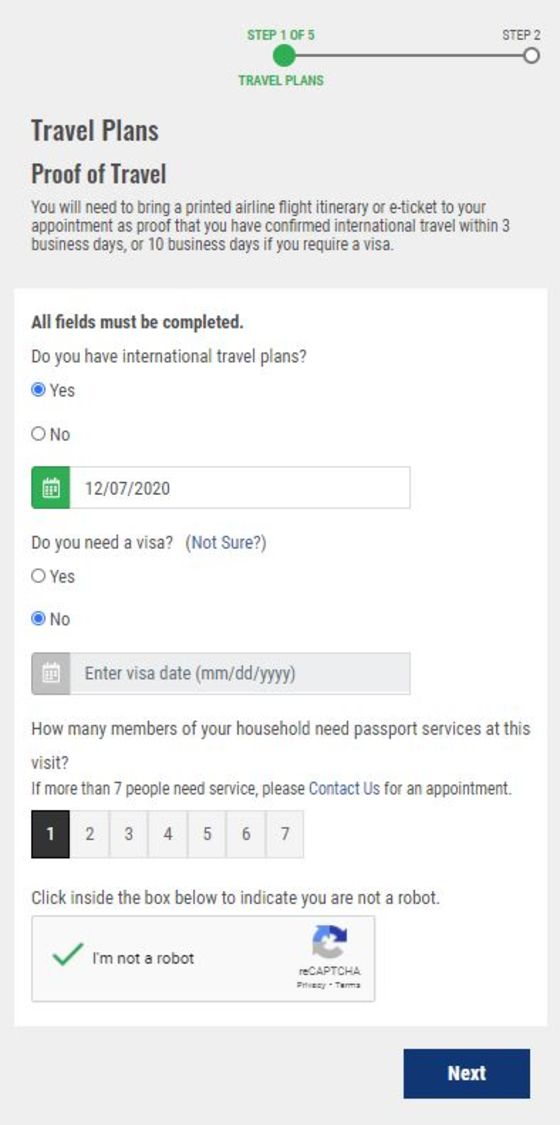The image is a mobile screenshot of a step-by-step checkout process in an app, likely for scheduling a visa or passport service appointment. At the top, there is a step navigation panel showing five steps, with step one highlighted in green, labeled "Travel Plans." Step two is not yet completed and appears in gray and white, connected to step one by a gray line.

Below this, under the heading "Travel Plans," the section "Proof of Travel" instructs users to bring a printed airline flight itinerary or e-ticket to their appointment as proof of confirmed international travel within three or ten business days, depending on the visa requirement. 

Users are prompted with the question, "Do you have international travel plans?" with "Yes" selected in blue, while "No" is unselected. Next to a green calendar icon, the date "12-7-2020" is displayed.

Another prompt asks, "Do you need a visa? (Not sure)," with "Not sure" being a clickable link. "Yes" is unselected, and "No" is highlighted in blue.

Further down, there's a section to specify the number of household members requiring passport services, with instructions to contact the provider for appointments exceeding seven people. The options range from one to seven, with "one" selected in a black box.

Users must confirm they are not a robot by clicking within a box. A checkmark appears next to "I'm not a robot," followed by a CAPTCHA icon depicted with gray, blue, and dark blue arrows forming a circular shape, labeled "reCAPTCHA privacy terms."

At the bottom, there is a blue "Next" button with white font.